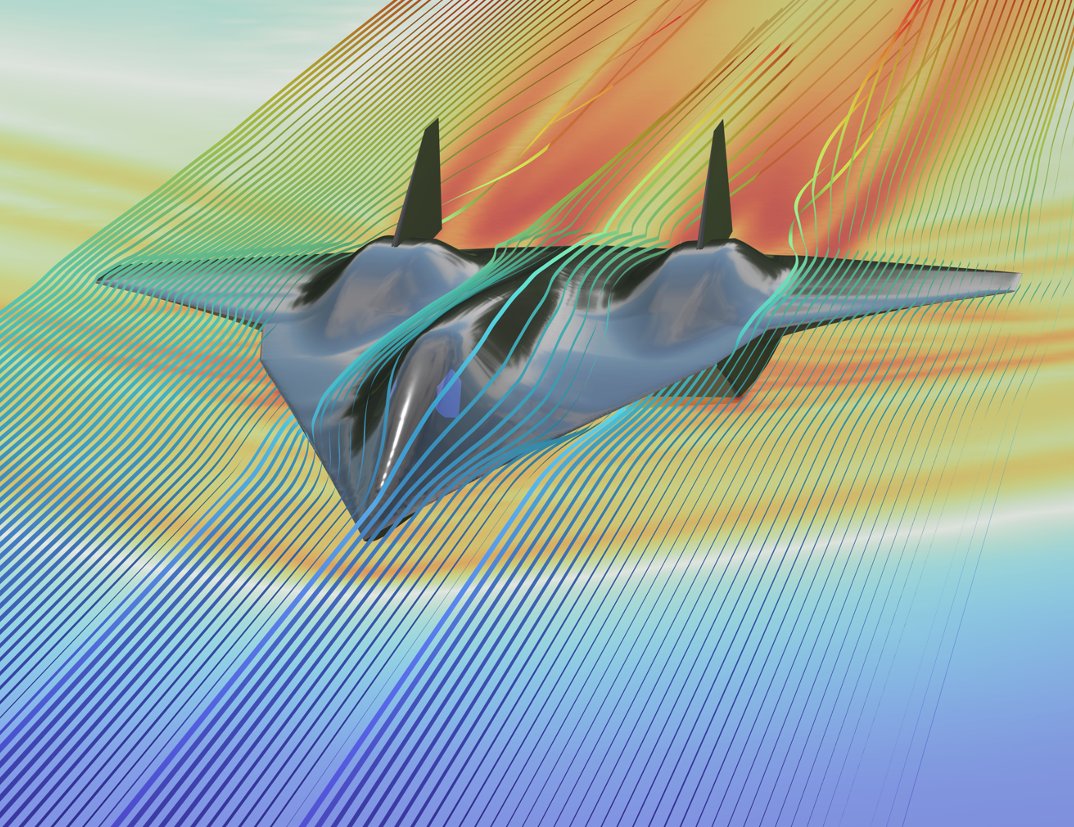The image depicts a digital rendering of a sleek, black military stealth bomber flying through a vivid, colorful background. The stealth bomber, characterized by its distinct rear fins and angular design, glides diagonally from the upper right to the lower left of the composition. Surrounding the aircraft are wavy, pencil-like lines and stripes of various colors, including blues that transition from dark to light, greens, aquas, yellows, reds, and oranges. These lines, reminiscent of wind tunnel aerodynamics, illustrate how airflow interacts with the aircraft, blending together where the plane disrupts them. The background is a striking mix of blues, yellows, oranges, and off-whites, adding to the artwork's dynamic and almost psychedelic appearance. The overall effect is a vivid visualization of the stealth bomber’s flight through turbulent, colorful air currents.